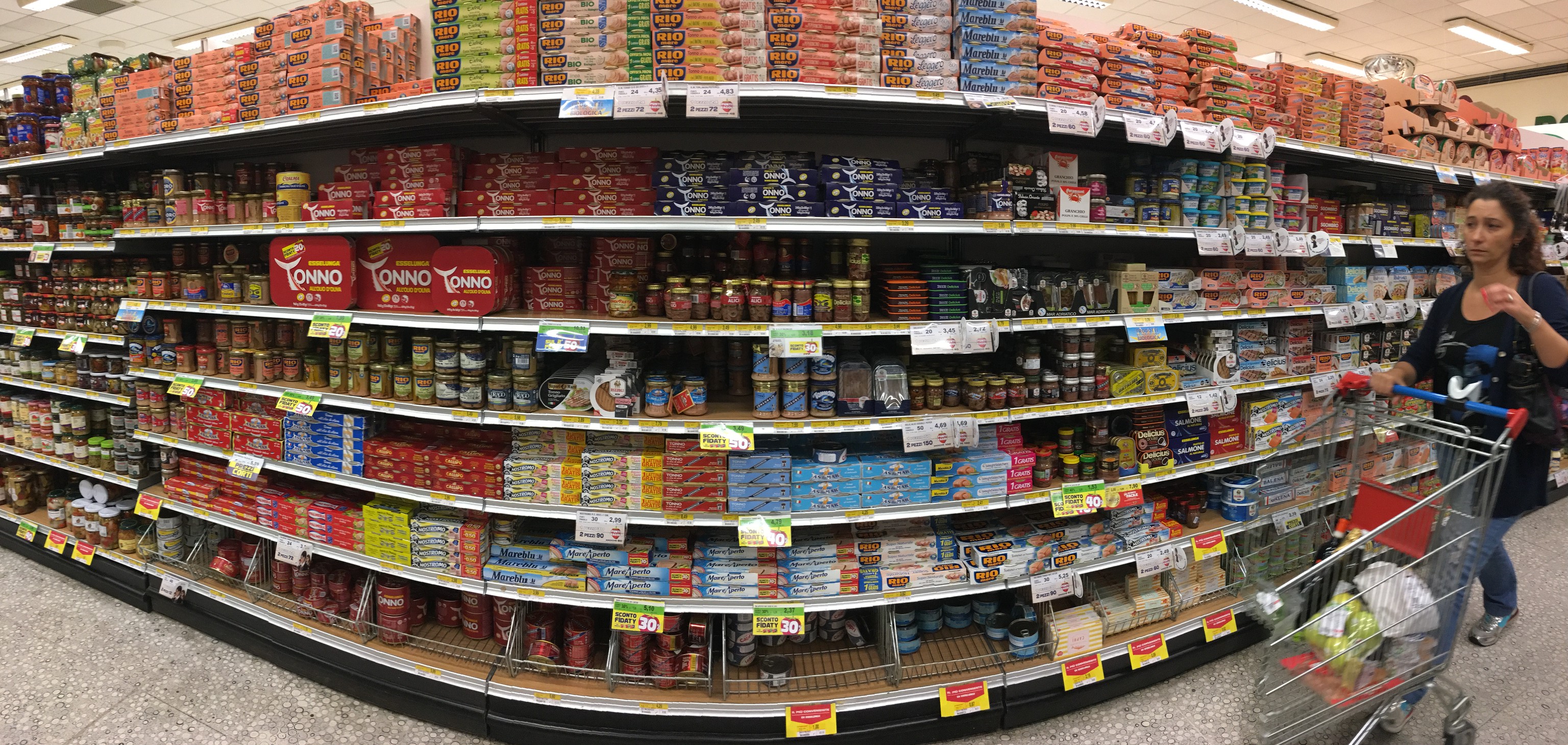In this rectangular photograph taken inside a supermarket, we observe an intriguing scene at a rounded corner of an aisle. Central to the image is a young woman pushing a shopping cart, though notably, the cart has been digitally altered. Specifically, the top or rear third of the cart is missing, as though it has been photoshopped out. The woman grips the blue handle of the cart, which contains various items, though the missing portion at the back is conspicuously absent.

Adjacent to her, the shelving along the aisle is stocked with items spanning approximately seven shelves high. At the lower levels, vibrant yellow and red tags indicate sale items, accompanied by white tags displaying prices. While some of the figures on these tags are discernible, the exact nature of the products remains unclear; they include boxes, cans, and glass jars with lids. On the upper left side, the top shelf features a branded product line named 'Rio', housed in long, multicolored boxes. The specific contents of these boxes are indistinguishable from the images on their packaging.